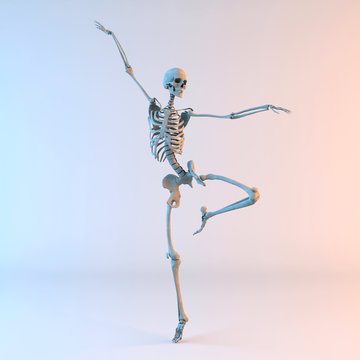The image features a digitally created human skeleton posed in an elegant, balanced stance reminiscent of a ballerina. The skeleton stands on its tiptoe with its left knee bent, its left arm extended outward, and its right arm elevated above its head. The background of the image transitions smoothly from a very light blue on the left side to a peach and muted orange on the right, blending into a mix of pastel shades. The skeleton is centrally positioned against this indeterminate backdrop, creating a striking and somewhat whimsical visual effect that could be interpreted in a variety of contexts, from educational to humorous.